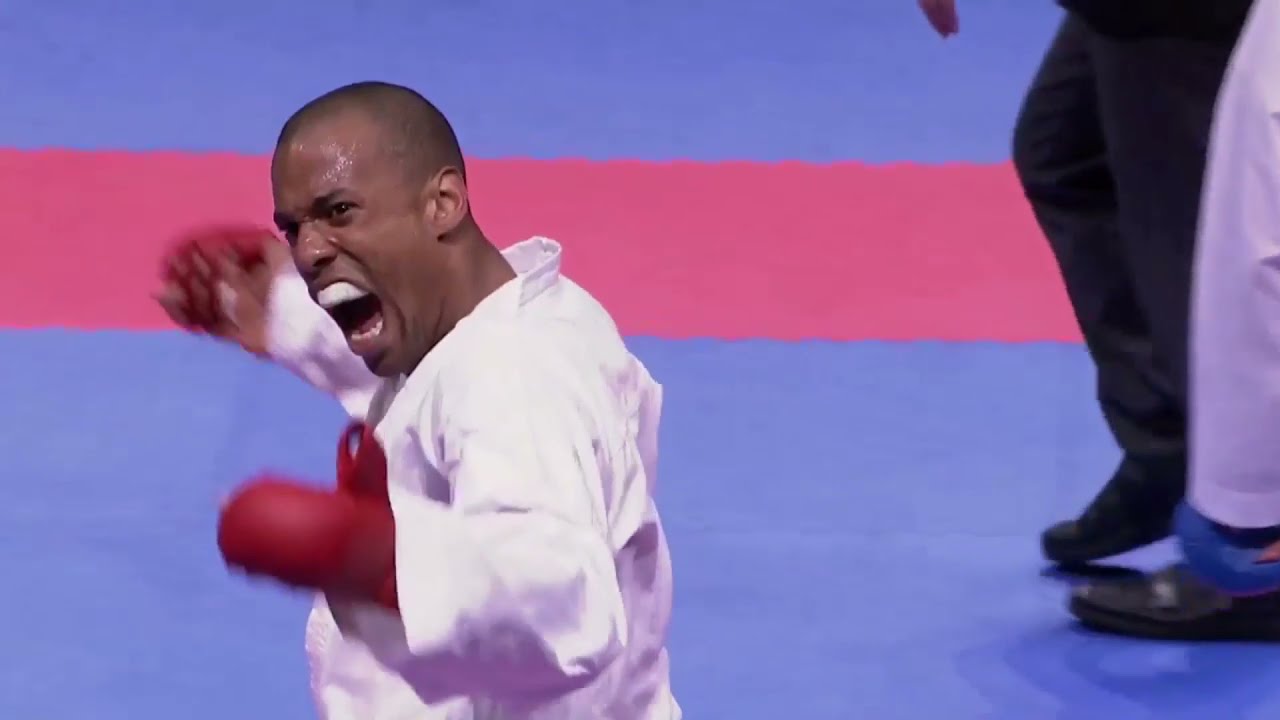The photograph captures an intense moment at a martial arts tournament set on a blue mat with a horizontal red stripe. Dominating the left side of the image is an African American man wearing a white gi, indicative of karate, with red mitts on his hands for punching and blocking. He is positioned with the left side of his body towards the camera, his mouth wide open to reveal a white teeth guard, giving the impression of yelling or letting out a celebratory scream. His arms are raised in a defensive or triumphant strike position, suggesting he may have just won his match. The background includes the lower half of two other participants on the right side of the image, one with white pants and the other with dark-colored pants, further highlighting the competitive atmosphere of the scene.